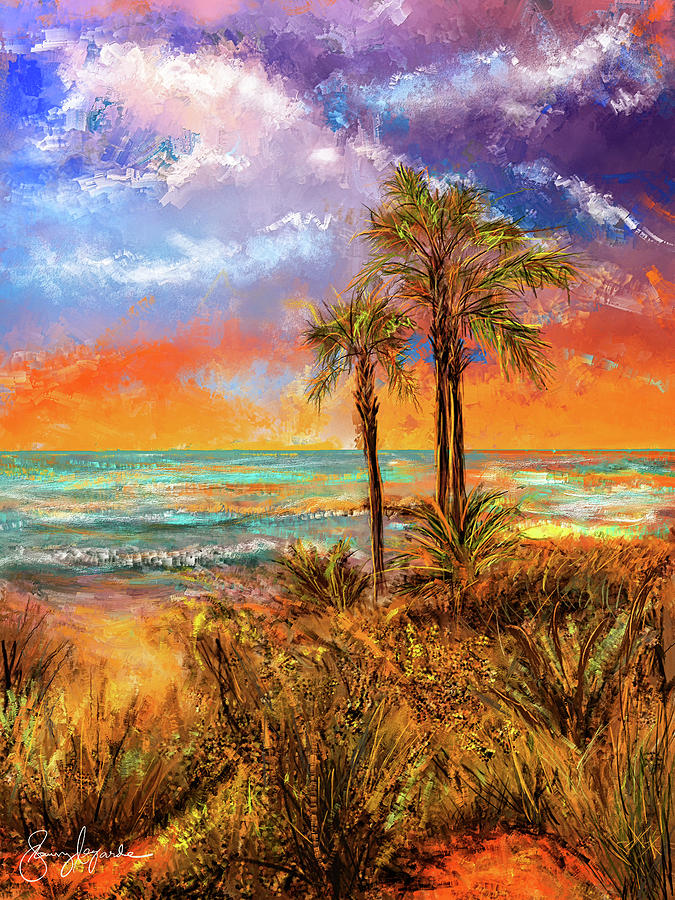The painting depicts a vibrant Florida beach scene. The sky transitions from a purply blue at the top to a mesmerizing mix of blue, white, and bright orange clouds near the horizon. The water below is a striking turquoise blue with patches of orange reflections, detailed with white brushstrokes mimicking rolling waves. In the foreground, the beach sand varies from a reddish hue near the grassy areas to a bright orange closer to the shore. Three prominent palm trees with black trunks and a mix of neon green and dark leaves stand tall near the center of the scene. Shorter green grasses are scattered around, adding to the lushness of the beach setting. The artist's white cursive signature is inscribed in the lower left corner, completing this intricate and colorful depiction of a coastal paradise.